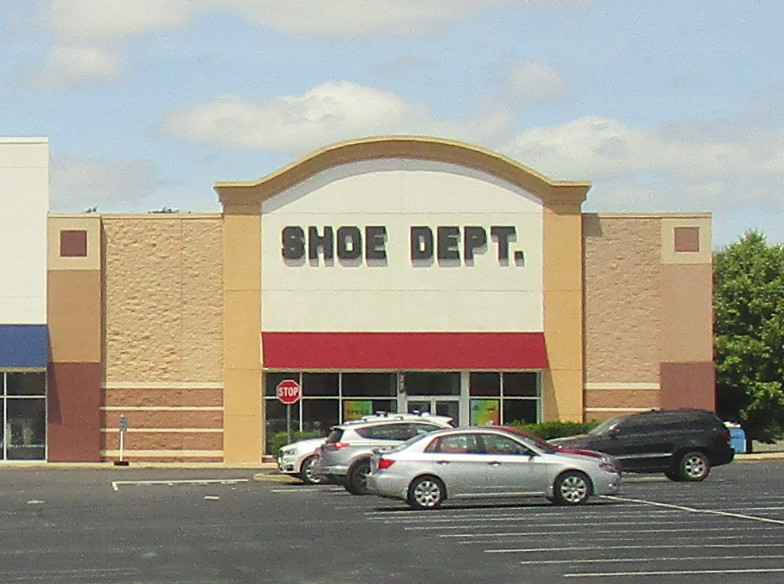The daytime outdoor photograph captures a bustling scene in bright sunlight, featuring a shoe department store set against a clear blue sky with drifting white clouds. The storefront of the SHU DEPT PERIOD store showcases a combination of dark and light tans and browns, with a distinctive curved roofline. The facade is adorned with a red awning above the entrance and is framed with rectangular glass panels outlined in white. Bold black letters spell out "SHU DEPT" on a white background above the entrance.

In the foreground, the parking lot is marked by white lines delineating the parking spaces, over a dark gray pavement. Four to five vehicles are visible: a silver sedan prominently facing right, a red car behind it, a gray SUV, and a black SUV. There is also mention of a possibly white vehicle. To the right, a green, fully-grown tree adds a touch of nature to the urban setting. Additionally, a stop sign is situated just beyond the parking area, emphasizing the orderly layout of the space. Adjacent to the shoe store is another establishment with a blue awning, hinting at a connected row of shops. Despite a slight graininess, the image maintains clear focus and detail.